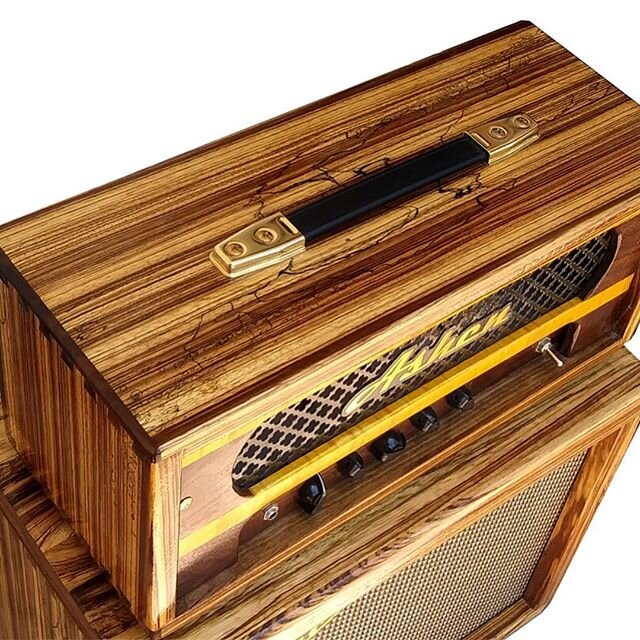This square-format color photograph offers an overhead view of an audio setup consisting of two stacked speakers encased in brown wood frames. On top sits a custom-made receiver featuring a black handle secured by brass fittings at each end. The receiver's rectangular top is angled from the bottom left to the top right, and its front panel features an elliptical cut-out with a mesh screen overlay. Staying true to meticulous craftsmanship, a gold logo with the scripted text "Ashen," spelled out as A-S-H-E-N, adorns the top of the receiver. Below the logo lies a gold strip, partitioning the controls, which include several black knobs aligned under the strip and a single silver switch positioned at the bottom right. The wooden casing of the underlying speaker matches the rich brown hue of the receiver, enhancing the cohesive visual appeal of the setup. The photograph's background has been removed, creating a floating effect against a white backdrop. The image is tightly cropped on the right, bottom, and left edges, lending a focus to the detailed, realistic representation of the audio equipment.